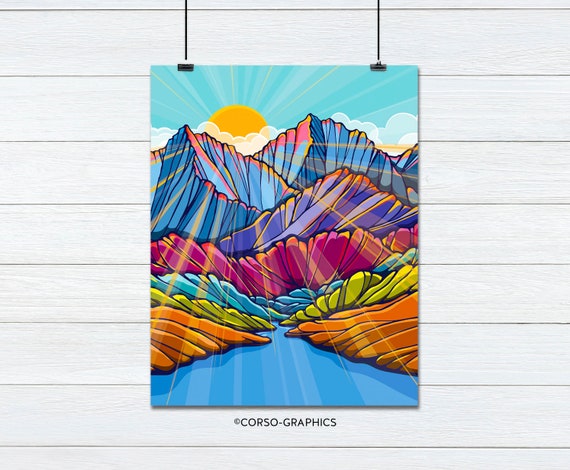This is a vibrant, colorful art piece showcasing a surreal outdoor landscape that appears to be either a drawing or a computer-generated image. The painting, which is in portrait layout and hangs on a white-paneled wall with horizontal wood siding, is suspended by two black strings attached to binder clips.

At the top of the image, a bright yellow sun with rays spreading outward is set against an aqua blue sky, dotted with some white clouds. The sun's rays peer through a V-shaped structure formed by craggy mountain peaks. The mountains are depicted in an array of vivid, unrealistic colors, including blue, purple, reddish-purple (cranberry), yellow, lime green, and orange. The edges of these craggy mountains feature tints of orange and yellow, contributing to the overall cartoon-like aesthetic of the scene.

In the lower part of the painting, a triangular blue lake extends from the bottom corners towards the center, enhancing the dynamic composition of the piece. The entire artwork is detailed with captions reading "Copyright Corso-Graphics" at the bottom in gray text. The vivid and diverse palette of colors—from purples and blues to reds, yellows, and greens—creates a lively and detailed depiction of an abstract, imaginative landscape.